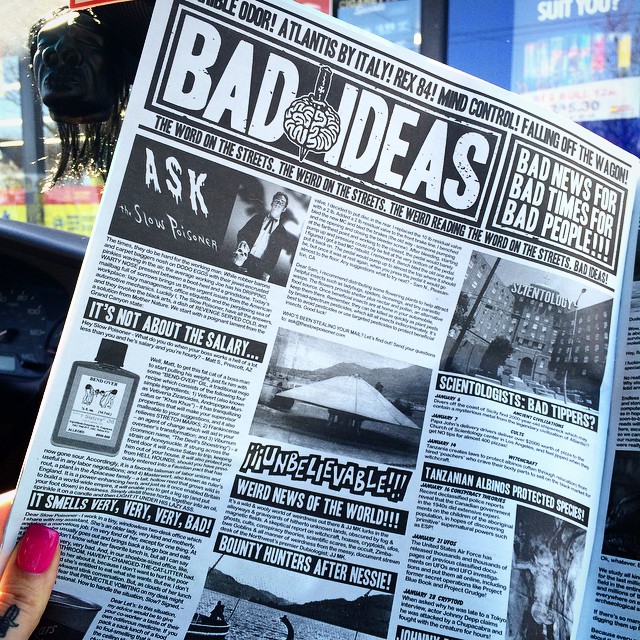A woman with a large pink nail and a small knife tattoo on her thumb is holding open a traditional black-and-white tabloid newspaper. The paper is spread open to the center page, which is cluttered with black-and-white photographs and text in multiple columns, though much of the text is blurry. Prominently, the top of the page bears a big, bold logo reading "Bad Ideas" with an illustration of a brain skewered by a knife. The chaotic headlines include: "Terrible Odor," "Atlantis by Italy," "Rex 84," "Mind Control," "Falling Off the Wagon," "Bad News for Bad Times for Bad People," "The Word on the Streets," "The Weird on the Streets," "The Weird Reading the World on the Streets," "It's Not About the Salary," "Smells Very, Very Bad," "Unbelievable," "Weird News of the World," "Bounty Hunters After Nessie," "Scientologists: Bad Tippers," and "Tanzanian Albinos Protected Species." The woman appears to be sitting outdoors, with a hint of a blue sign saying "Sun 2" visible in the background. This newspaper mimics the sensational style of publications like the National Enquirer, filled with bizarre and outrageous stories.